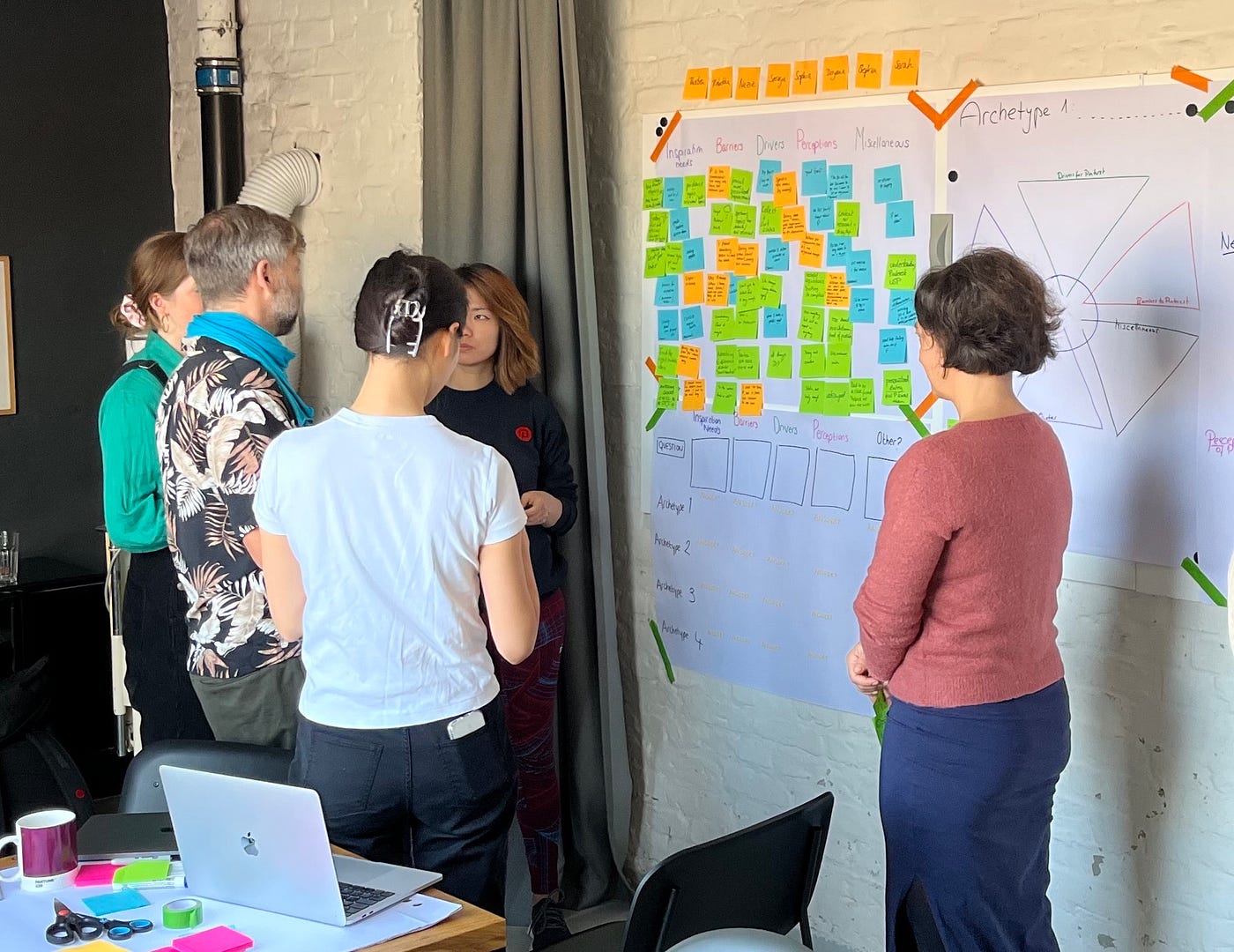In an indoor office setting, this photograph captures five people engaged in a brainstorming session in front of a white-painted brick wall. The focal point of the image is a large whiteboard covered with multicolored square-shaped post-it notes—blue, green, and orange, each adorned with text. Just below the sticky notes are a series of diagrams and drawings of five boxes. Additionally, there's a paper affixed to the wall using green and orange tape, displaying a pinwheel-like design labeled "Archetype" with five parts or fins.

Among the five individuals, four have their backs to the viewer, while one faces the camera. The man facing forward wears a Hawaiian pattern tan on a black background and a blue scarf. One woman, wearing a green shirt with black overalls, is turned away. The woman in the foreground sports a white t-shirt, dark pants, and a hair clip in her brown hair. The woman closest to the whiteboard has distinctive red hair, is clad in a black long-sleeved shirt with a red dot on it, and black pants. The farthest right individual, dressed in a pink long-sleeved sweater and blue skirt, has brown hair and faces toward the group.

Behind them is a table cluttered with various items, including a laptop, an Apple computer, scissors, post-it notes, and a mug, with a couple of chairs positioned nearby. A gray curtain is also visible in the background. The scene conveys a collaborative atmosphere, as the group appears deeply engaged in planning or designing something together.